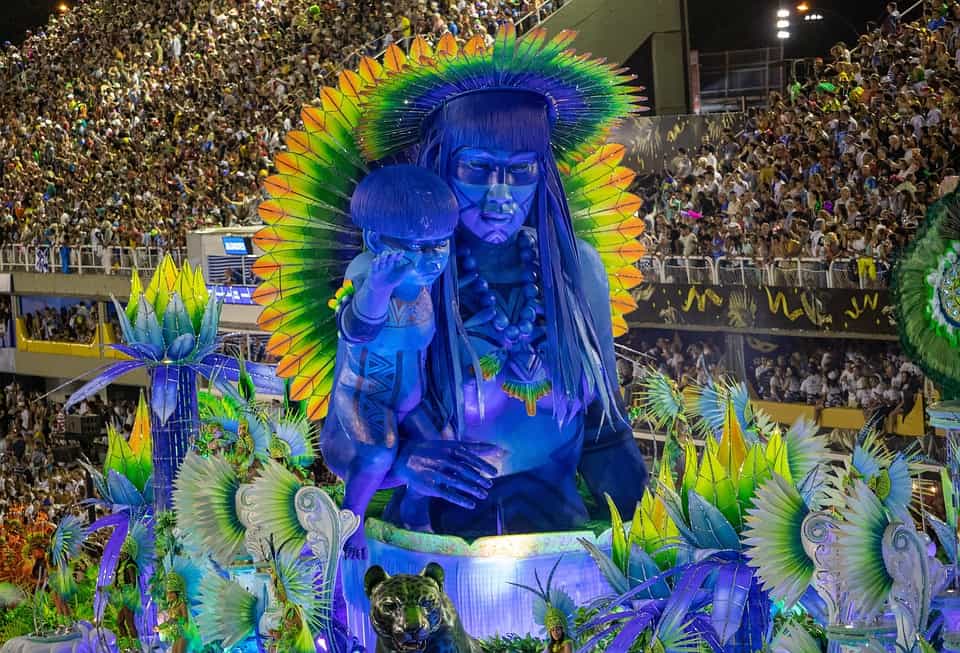In the image, a vibrant parade is underway, likely in a large, packed stadium filled with three rows of bleachers teeming with thousands of spectators. The focal point is an elaborately decorated float featuring a striking blue statue of a Native American figure adorned with a green and yellow feathered headdress. The figure has long blue hair, blue bangs, and distinctive blue markings around the eyes. It wears a large clunky wooden bead necklace and holds a similarly blue child with matching blue eye masks and bangs on its raised arm.

The float itself is a burst of colors, majorly featuring shades of green, blue, orange, and yellow, intertwined with elaborate decorations like green and white leaves and possibly a gold jaguar on one side. The scene is rich with additional colorful floats and accessories, heightening the celebratory atmosphere. The entire event is brimming with vivid shades of light blue, fuchsia, black, gray, and white, with the exuberant crowd in the bleachers keenly watching the parade's progression.